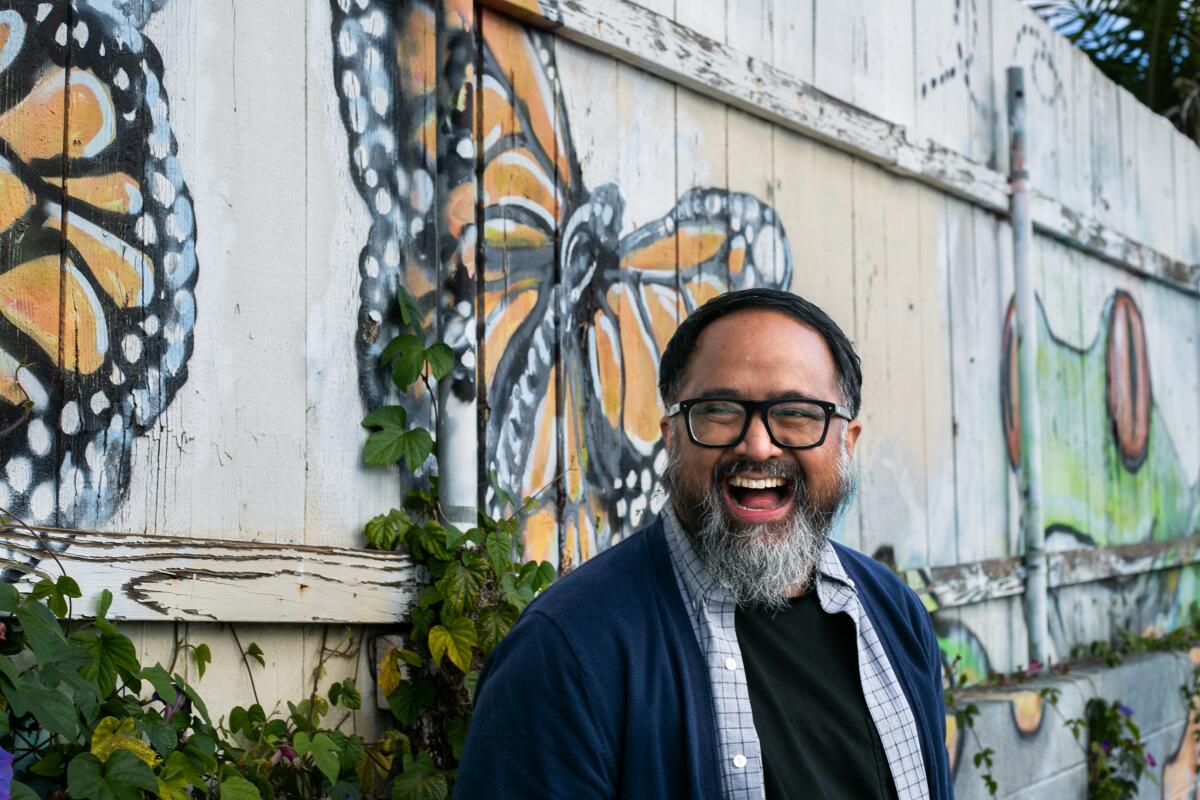In the daytime outdoor image, a man is prominently positioned in front of a partly white-painted wooden fence that spans the background from left to right, mounted above a cinder block base. This fence features vibrant graffiti art, with two black and orange butterflies on the left and a frog on the right. Additionally, green foliage or vines climb up one of the fence posts, contributing to the lively scene. The man, who has black hair, a scraggly black and gray beard that extends to a silver goatee, and a wiry mustache, is captured in a joyful moment, laughing heartily with his mouth wide open, teeth, and tongue visible. His head is slightly turned to the right. He wears glasses, a black t-shirt, a checkered button-down shirt, and a blue sweater layered over it. A subtle, small cap that appears to be a Jewish kippah adorns his head, adding further character to his appearance. The various colors present, including yellows, blues, blacks, grays, greens, tan, red, and lime green, enrich the overall vibrant and textured composition of the photo.